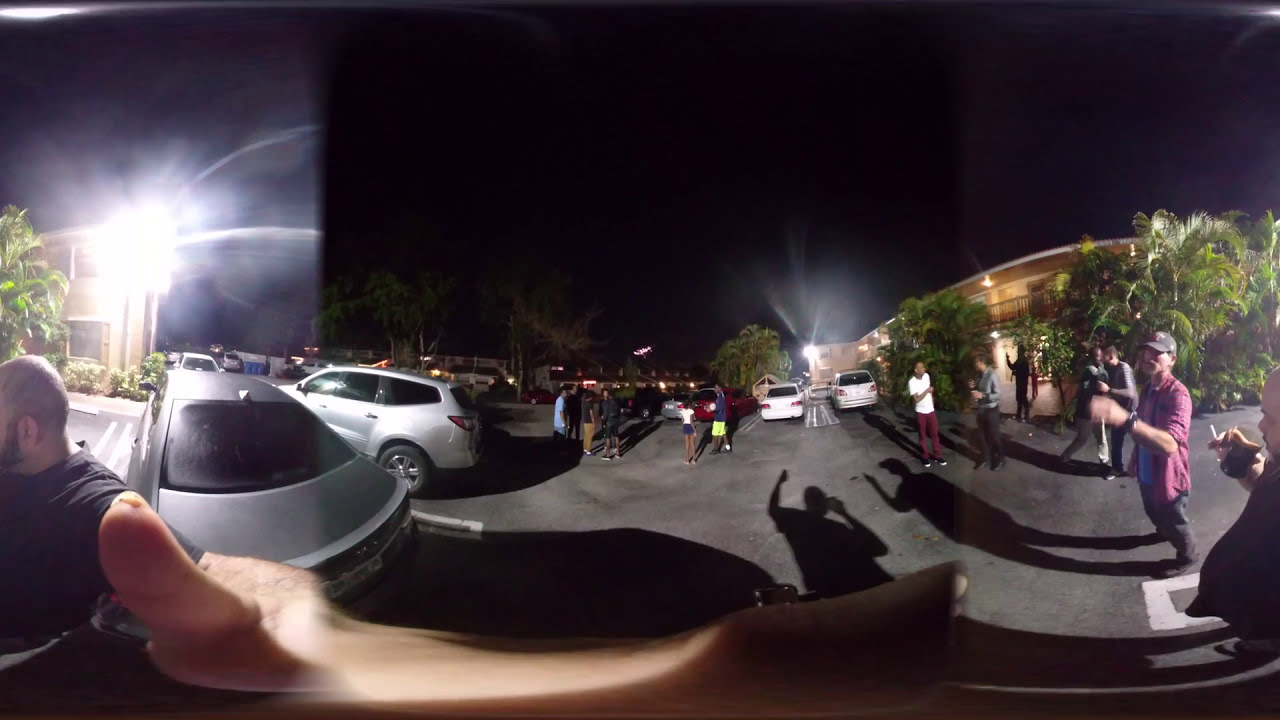The image depicts a bustling nighttime gathering in a parking lot, possibly outside a hotel, apartment building, or mall. Approximately 20 people, comprising both men and women, are scattered around the lot where about 15 cars are parked. With a sky that is pitch black, the setting is illuminated by various light sources casting shadows of the cars and people. Towards the left of the image, a man with his back to the camera holds a flashing camera, drawing the attention of the onlookers. In the foreground and middle sections, the crowd appears engaged, possibly recording or observing an event, adding to the dynamic atmosphere. On the right-hand side, a group of seven to eight people congregates near green trees with palm branches. Among the spectators, a man in flashy red pants and a white shirt, as well as another bald man, can be seen. The photo captures a scene filled with anticipation and curiosity, suggesting that a notable activity or commotion is happening towards the left of the frame.